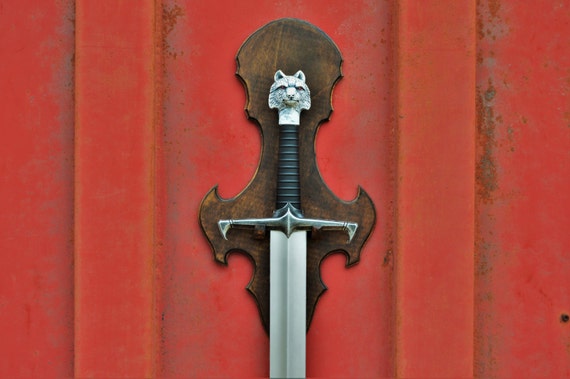A full-color, square photograph taken outdoors showcases a red corrugated metal wall, speckled with rusty spots, serving as the backdrop. Mounted on this weathered surface is a wooden base from which a sword hangs. The sword's handle is black, featuring a wrist guard to protect the wielder. The handle culminates in a silver wolf's head, complete with intricately detailed ears, eyes, and nose. Visible beneath the handle, about six inches of the blade extend downward, disappearing off-screen. The image contains no text, people, or animals, focusing solely on the striking juxtaposition of the sleek sword against the rugged, rusty red wall.